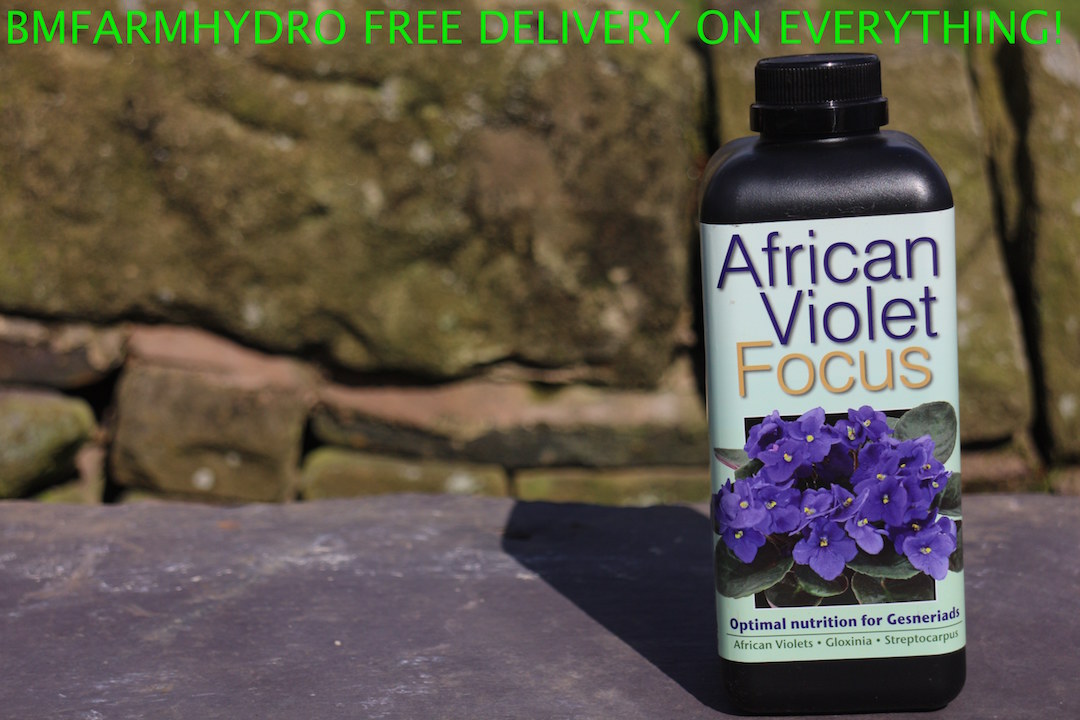This advertisement showcases a product from BM Farm Hydro with the headline "FREE DELIVERY ON EVERYTHING!" in neon green, capital letters at the top. The product, displayed prominently in the foreground, is a sizeable black plastic bottle with a white label depicting vibrant, blooming African violets. The label reads "African Violet Focus" and indicates that it provides "Optimal Nutrition for Gesneriads". The bottle is placed on a concrete surface with an out-of-focus rock wall in the background, adding a rustic touch to the presentation.